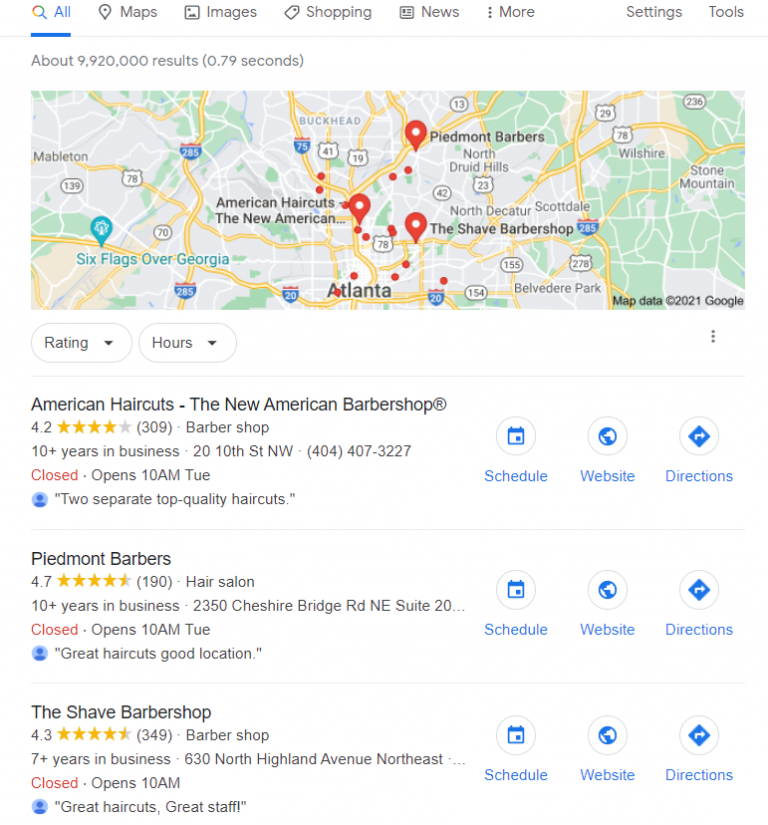The image is a vertically-oriented screenshot of a Google search results page. At the top, the navigation bar displays options such as 'All,' 'Maps,' 'Images,' 'Shopping,' 'News,' 'More,' 'Settings,' and 'Tools,' written in gray, except 'All,' which is highlighted in light blue, indicating it is the selected tab. Below the navigation bar, the text indicates that there are approximately 9,920,000 results found in 0.79 seconds.

The main section of the image displays a Google Map centered around Atlanta, marked by three red location pins. Each pin corresponds to a different barber shop. Directly beneath the map, two drop-down menus labeled 'Rating' and 'Hours' allow for further filtering of the search results.

The first search result is 'American Haircuts - The New American Barbershop.' The second result is 'Piedmont Barbers,' and the third is 'The Shave Barbershop.' Each listing includes the business’s rating and operating hours. On the right side of each listing are blue buttons labeled 'Schedule,' 'Website,' and 'Directions,' which provide quick access to each function specifically for the respective barbershop.